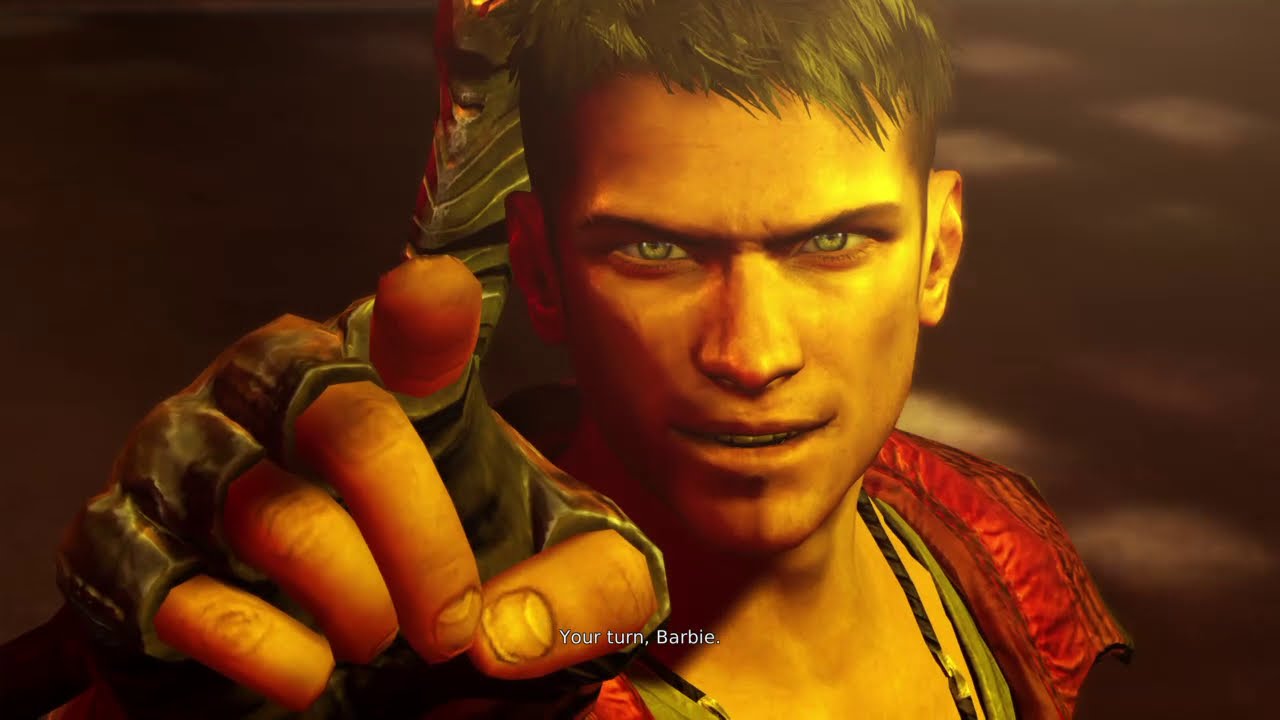The image is a detailed, animated scene, possibly from a video game. It features a male character with blondish-brown hair and a tan complexion, standing with his right shoulder closer to the camera and his head turned to look directly at it. He is wearing medieval-style attire, including a red vest or shoulder pad, a leather necklace, and a hilt of a sword that appears to be silver or gold, protruding from his back. The man is equipped with leather fingerless gloves, and his right hand is extended towards the camera, pointing with the index finger capped with red plastic. The scene is predominantly dark on the left side, with hints of light on the right, making it unclear whether it takes place indoors or outdoors. Overlaid text at the bottom of the image reads "Your turn, Barbie" in white font, suggesting a competitive or interactive scenario within the game.